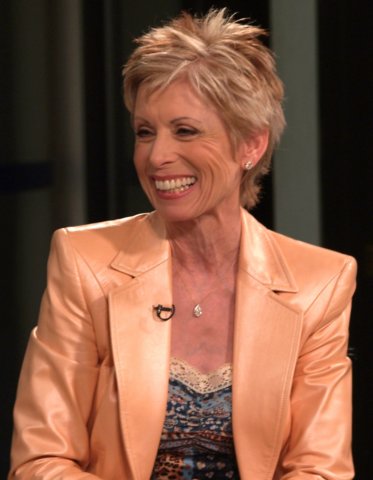The photograph depicts an older woman with short, spiky blonde hair styled into a pixie cut, slightly sticking up at the top. She is wearing a light, shiny orange suede jacket, which has been described by some as cream-colored leather, and a patterned low-cut shirt that combines blue and red hues adorned with white lace at the top. Around her neck is a silver necklace featuring a teardrop pendant. Her head is turned to the left as she faces the camera, revealing a broad, toothy smile with her eyes partially closed, highlighting some wrinkles around her cheeks. A microphone is clipped to the center of her jacket, suggesting she might be participating in a televised interview. The background is blurred but shows a shadowed wall and a bit of dark gray, adding a sense of depth to the image.